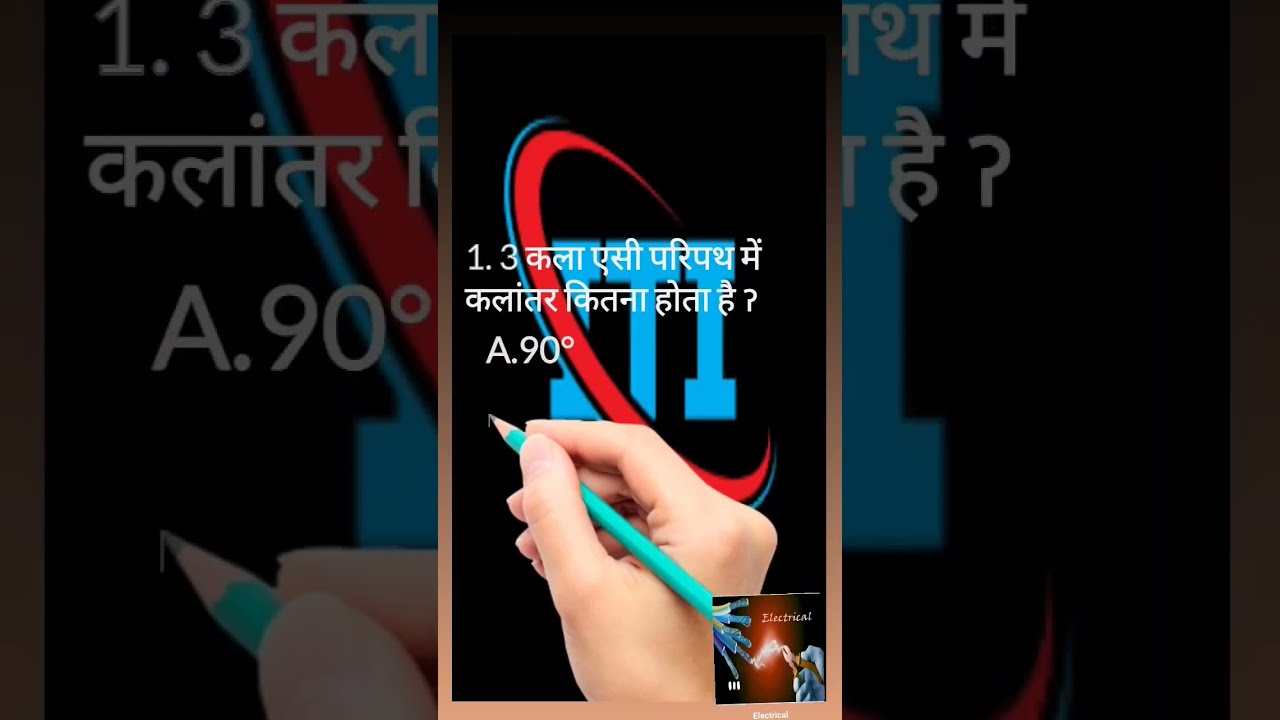In this image, a hand is prominently featured at the bottom center, holding a blue coloring pencil. The central part of the image showcases a logo that consists of a circular design encircling a symbol, possibly in Arabic script. Above the hand, there is an intricate mix of text, all in Arabic, along with additional numerals "1.3" and "A.90". The overall background of the image features colors such as black, blue, red, white, light blue, orange, and tan. A smaller, barely visible logo is positioned at the bottom right corner. The image appears to be a screenshot taken from a mobile device, likely from an app like TikTok or Instagram.